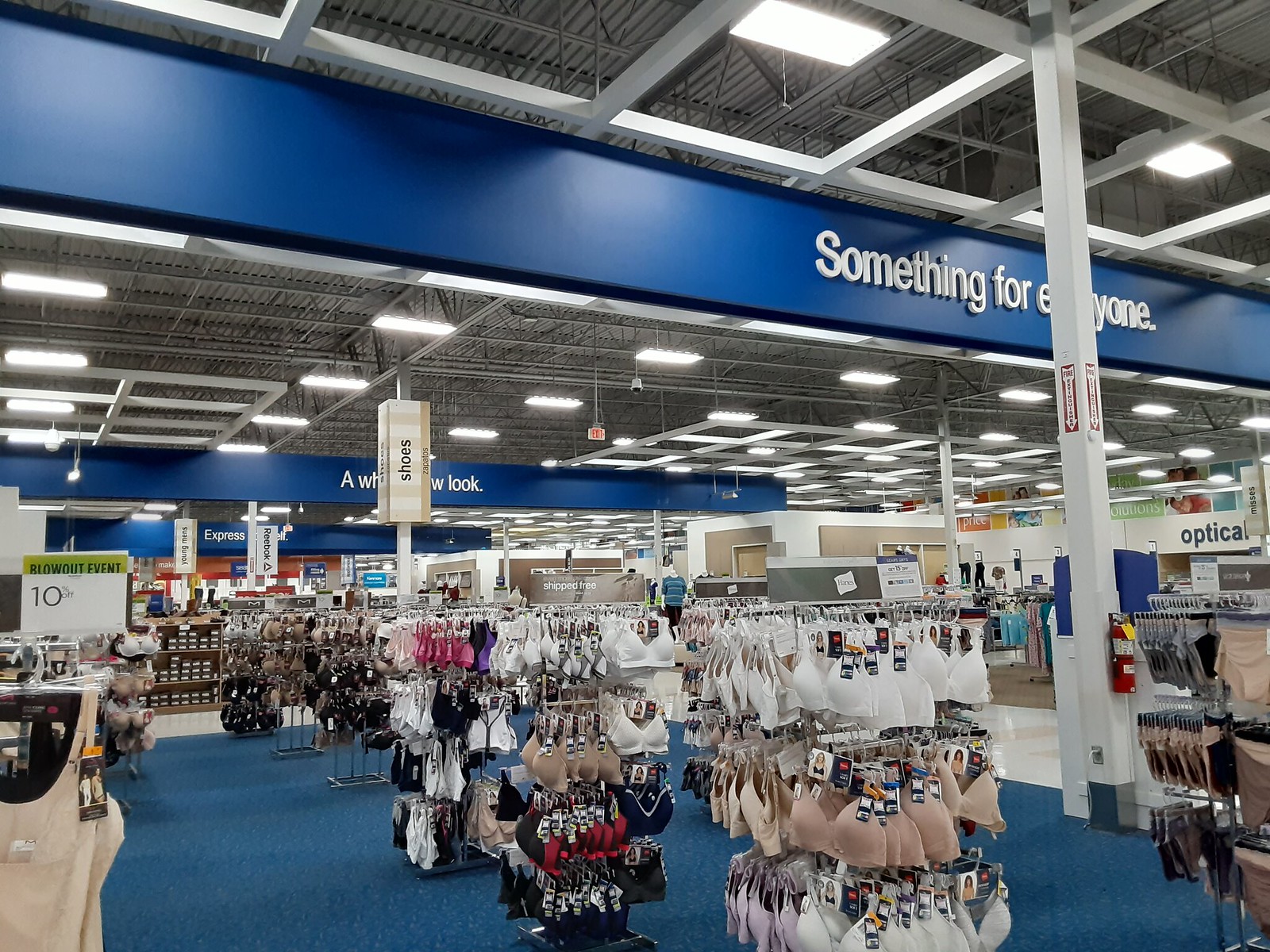This image depicts the interior of a large department store, visually reminiscent of a Walmart due to its dark blue and white color scheme, though no definitive Walmart signage is visible. The store features a vast, high-ceiling space resembling an aircraft hangar, with metallic piping, security cameras, and fluorescent lighting adorning the ceiling. The foreground showcases the intimates section, with racks of bras, camisoles, and underwear prominently displayed. Among the signage, one reads "C'est Blanc event," offering a "10% off" discount. A "Blowout event" sign is also noticeable near some camisoles. To the right, there's a post with a fire hydrant and signs indicating the optical department in the background. On the left, there is a section for shoes, indicated by a Reebok sign and visible shelves stacked with boxes. An overarching blue sign with white lettering reads "something for everyone," encapsulating the store's wide array of offerings.